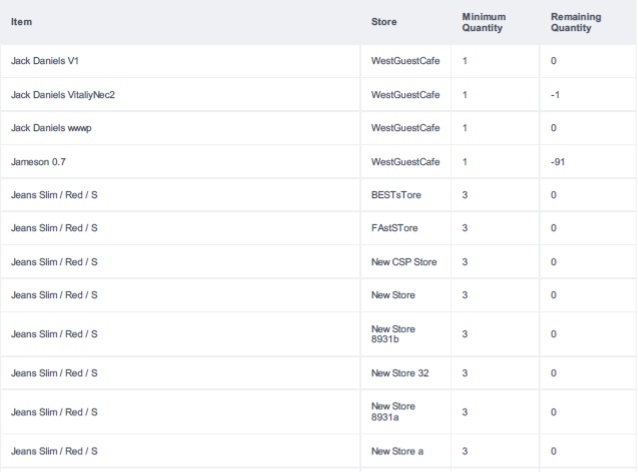This detailed descriptive caption provides an organized and comprehensive overview of the stock status captured in a screenshot of a webpage from multiple stores. 

---

In the screenshot, several items are listed along with their corresponding details, including the store name, minimal quantity, and remaining quantity. The background of the page is white, with all the text in black, neatly arranged in separated brackets for each category. 

1. **Jack Daniels V1** at West Guest Cafe:
   - Minimum Quantity: 1
   - Remaining Quantity: 0
   
2. **Jack Daniels Vitality Nectar** at Westgate Cafe:
   - Minimum Quantity: 1
   - Remaining Quantity: -1

3. **Jack Daniels WWP** at West Guest Cafe:
   - Minimum Quantity: 1
   - Remaining Quantity: 0
   
4. **Jameson 0.7** at West Guest Cafe:
   - Minimum Quantity: 1
   - Remaining Quantity: -91

5. **Gene Slim Red S**:
   - At Best S Store:
     - Minimum Quantity: 3
     - Remaining Quantity: 0
   - At Fast Store:
     - Minimum Quantity: 3
     - Remaining Quantity: 0
   - At New CSP Store:
     - Minimum Quantity: 3
     - Remaining Quantity: 0
   - At New Store:
     - Minimum Quantity: 3
     - Remaining Quantity: 0
   - At New Store 8931B:
     - Minimum Quantity: 3
     - Remaining Quantity: 0
   - At New Store 32:
     - Minimum Quantity: 3
     - Remaining Quantity: 0
   - At New Store 8931A:
     - Minimum Quantity: 3
     - Remaining Quantity: 0
   - At New Store A:
     - Minimum Quantity: 3
     - Remaining Quantity: 0

This stock list showcases the inventory status for various stores, indicating that most items are either out of stock or have negative quantities, suggesting a possible need for restocking or inventory adjustments.